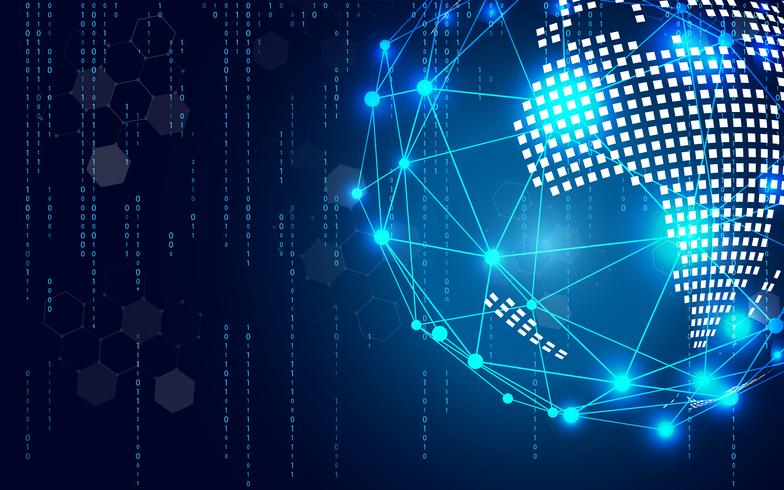The image depicts a striking digital rendering of a stylized Earth on a dark background that transitions into a brighter gradient toward the right. The backdrop is a mix of faint, translucent gray and dark blue hexagons, interspersed with binary code of zeros and ones streaming vertically like rain. On the right side of the image, a globe comprised of iridescent blue points and connecting lines represents planet Earth. Tiny white squares outline the continents, with Africa prominently visible and portions of Europe and the Middle East discernible above it. Bright blue nodes mark larger cities or key connecting points on the globe. The overall effect is of a mesmerizing, interconnected digital world, seamlessly integrating geometric patterns and binary streams.